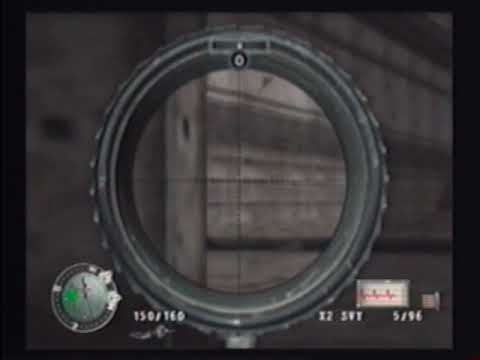The image is a blurry, black-and-white screenshot from a video game that depicts a war-torn or bombed stone building. The building, primarily gray, appears to be made of stone and concrete blocks, with significant portions crumbling to rubble, indicating severe destruction. To the left, an adjacent building made of large concrete blocks is visible. The bottom part of the image shows a character standing in the center, facing away from the camera and carrying a backpack or bag, blending into the deteriorating stone walls behind them. The bottom left corner features a compass-like circular graphic with a faint green color, and a briefcase icon with unreadable numbers underneath. The bottom right corner shows a number, likely a score, reading 57,160. The entire image is surrounded by a black border.